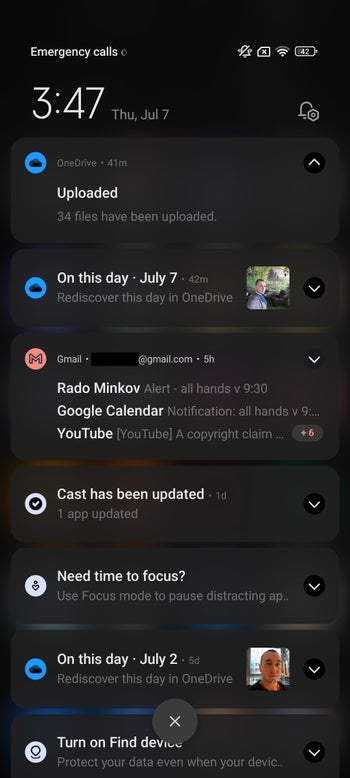Here's a detailed and cleaned-up caption for the image:

---

The image is a screenshot from an Android device, specifically capturing the contents visible after pulling down the notification shade in dark mode. The screen displays the time as 3:47 PM on Thursday, July 7th. The notifications fill the entire screen, starting with two from OneDrive. The first OneDrive notification, timestamped 41 minutes ago, informs the user that 34 files have been uploaded. The second OneDrive notification features a thumbnail image depicting a person in a natural setting and reads "On this day, July 7th, rediscover this day in OneDrive."

Below the OneDrive notifications, there is a cluster of Gmail alerts marked with the red Gmail logo. These include a message from Rydel Minkov regarding an "alert all hands V930," followed by a Google Calendar notification about the same event. Additionally, a YouTube notification mentions a copyright claim on one of the user's videos, indicating a potential copyright strike. The Gmail section also indicates there are six more unread messages with a "+6" in red.

Further down, the screenshot includes a few more app notifications, but they are not detailed in the description.